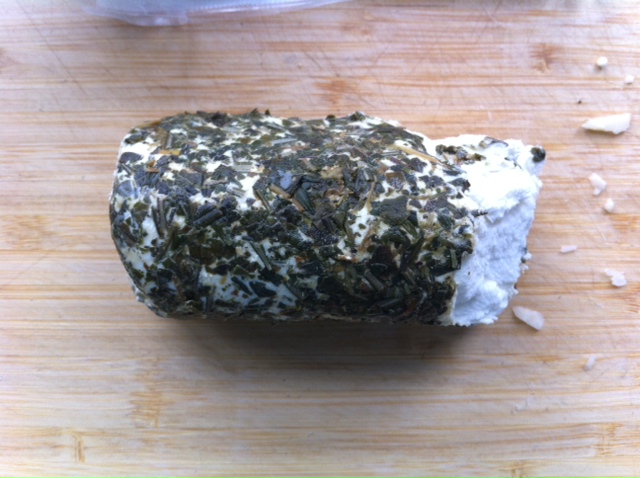The image depicts a cheese log coated with a blend of dark-colored herbs and seasonings, primarily dark green, brown, and black. The cheese itself is white, and a piece has broken off on the right side, revealing more of the white interior. This breakage has left small white crumbs scattered around the log. The cheese log rests on a light brown wooden surface, where the wood grain is visible. At the top left corner of the image, there is a glimpse of what appears to be a plastic container.